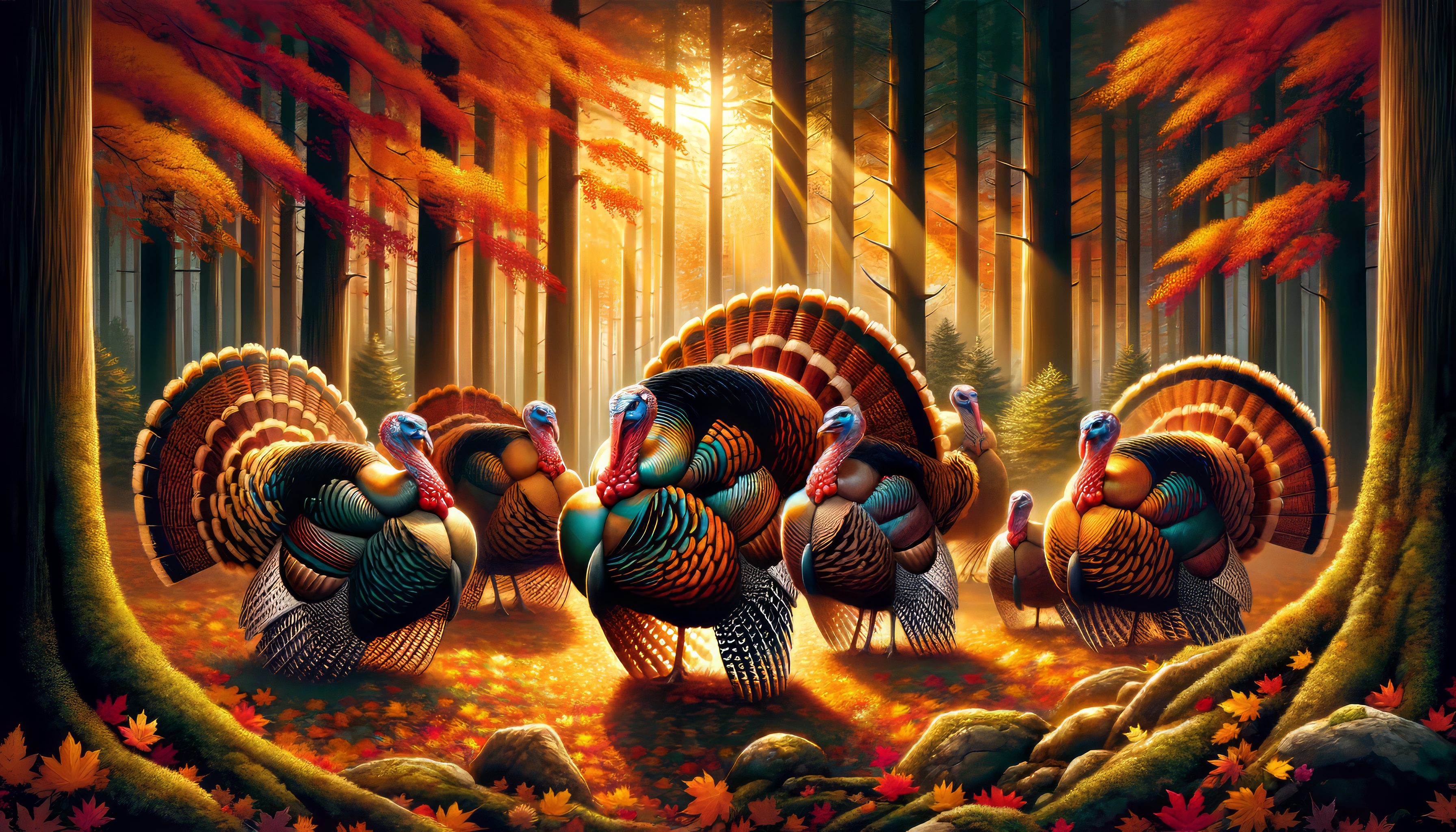In this detailed and slightly cartoony AI-style image, a group of seven turkeys is depicted standing in a North American autumn forest. The largest turkey is in the middle, with the others varying in size around it, including one small turkey that appears to be a juvenile. The turkeys have striking features: they possess large, fan-like feathers in shades of dark orange, black, and beige, with their bodies displaying a mix of turquoise and burnt orange. Their necks are a vivid red, faces are blue, and they have orange beaks, all of which lend them a serious and engaged appearance, as if preparing for a confrontation. The forest setting enhances the scene, with tall brown trees adorned with a mix of green, red, and orange foliage. The ground is carpeted with fallen leaves, contributing to the overall autumnal ambiance. Sunlight filters through the trees, illuminating the vibrant colors of the leaves and enhancing the picturesque quality of the scene.